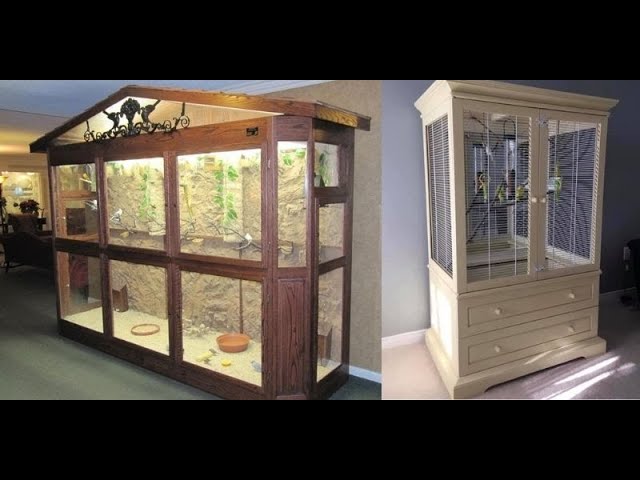The image features two adjacent photographs, each showcasing different yet intricately detailed wooden bird cages that resemble cabinets. The cage on the left is larger with an oak, gable-roofed frame featuring three large doors and elegant wrought iron decoration at the top. Its interior is meticulously arranged with terracotta water bowls and gravel on the floor, creating a refined homey environment. The right-side cage, narrower and taller, resembles an antique two-door china cabinet—repurposed with bird cage wire—retaining its original drawers at the bottom and glass windows. Both cages display a variety of colors including browns, tans, and grays, and the juxtaposition emphasizes their unique designs while highlighting their shared function as bird habitats. The image, taken indoors against a blue wall with carpeted flooring, shows no text and is framed with black borders at the top and bottom.